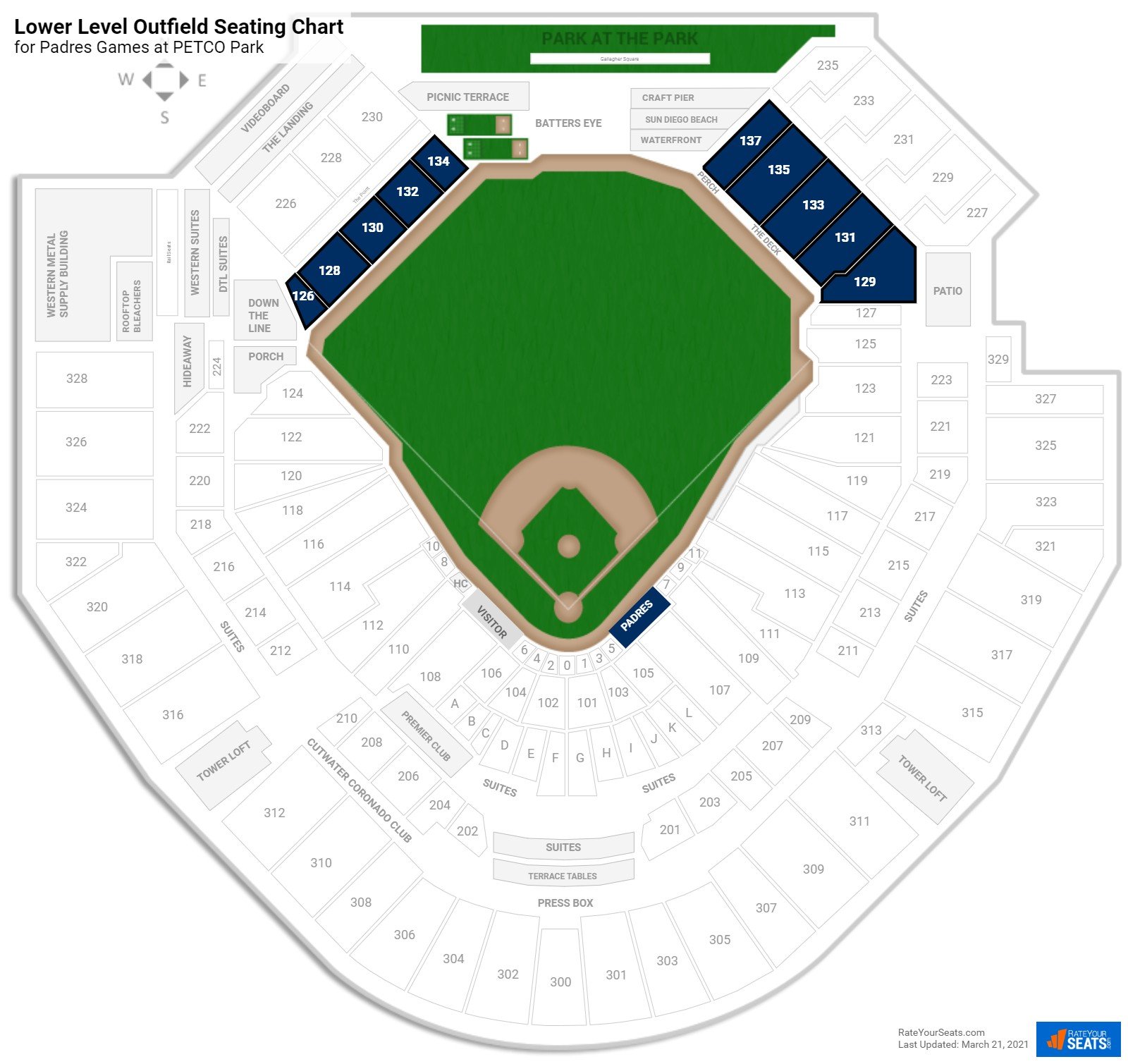This image showcases a detailed seating chart for Padres games at Petco Park, specifically focusing on the lower level outfield seating. The photo is set against a white background with a subtle gray border outlining the stadium's perimeter. 

At the center of the sketch is the baseball field, vividly highlighted in green and brown to represent the grass and the infield, outfield, and warning track. Flanking the field on both sides are two sets of blue-highlighted boxes: the left set ranges from sections 126 to 134 with 5 sections, and the right set ranges from sections 129 to 137 with another 5 sections, likely indicating the outfield seating areas.

Prominently on the right side between first and third base is a blue icon labeled "Padres," marking the home dugout, with the visitors' dugout situated to the left. Adjacent to the field are areas marked in green, signifying the bullpens.

To the top of the image, there is a green expanse named "Park at the Park," providing an additional scenic feature of the stadium. In the upper-left corner, the title "Lower Level Outfield Seating Chart for Padres games at Petco Park" is displayed, accompanied by a compass indicating cardinal directions (North, East, West, South).

Surrounding the highlighted sections are numerous other unhighlighted boxes and seating areas, representing parts of the stadium not included in the lower level outfield seating.